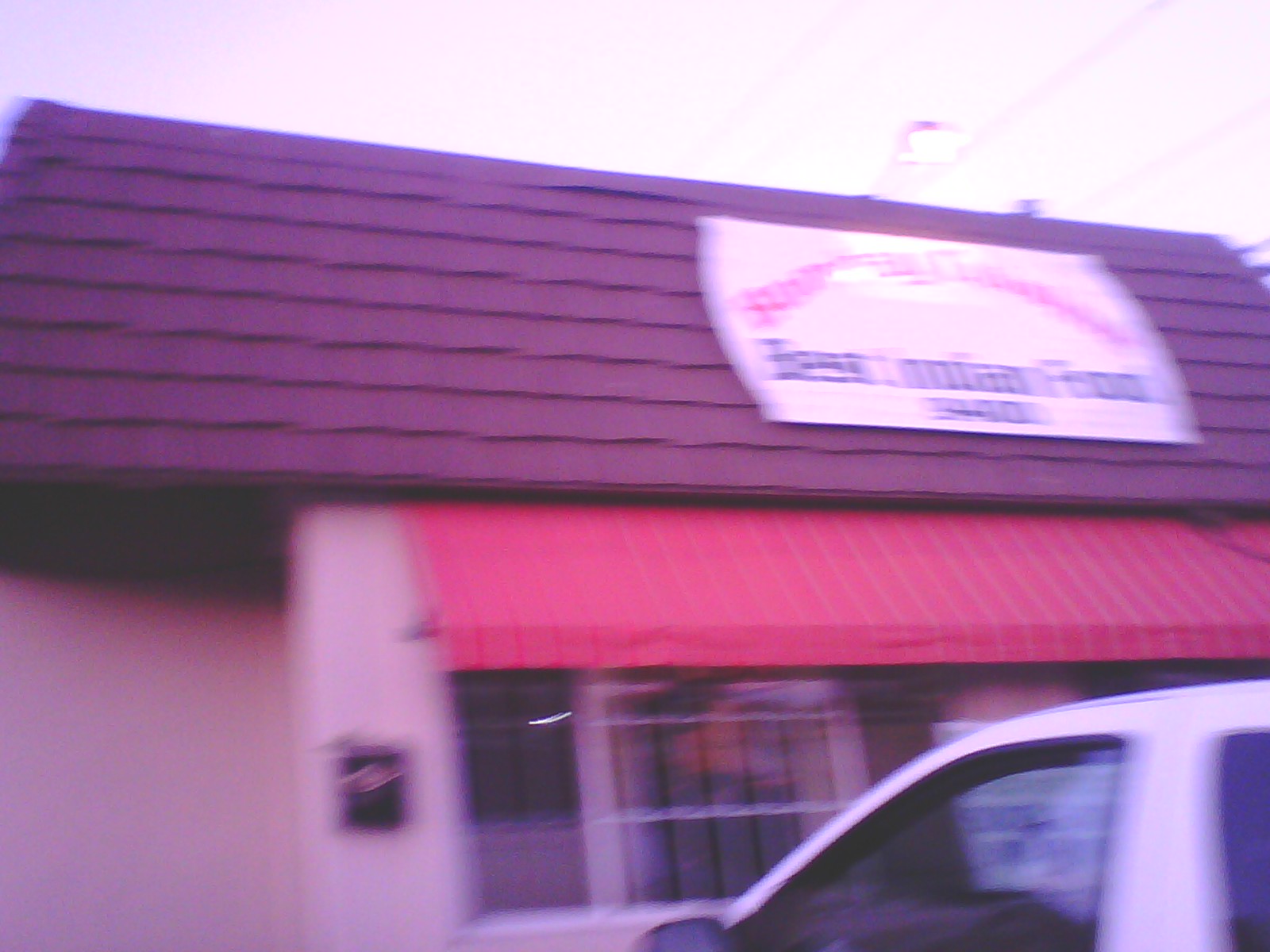This color photograph depicts a slightly blurry, non-American restaurant with a distinctive red shingled roof that ascends sharply. The sky above the establishment appears white or pink, indicating possible snowfall in the area. A streetlight and power lines are visible above the building. The storefront is painted pink, and there's a red sunshade over the barred windows with white bars. A white vehicle, either a car or a truck, is parked in front, partially obscuring a sign visible through its windshield. A black mailbox stands near the front of the store. The building features a veranda with vertical pink lines and a mirrored tile roof, and a sign that's white with red and blue colors, though the text is unreadable due to the image's blurriness.